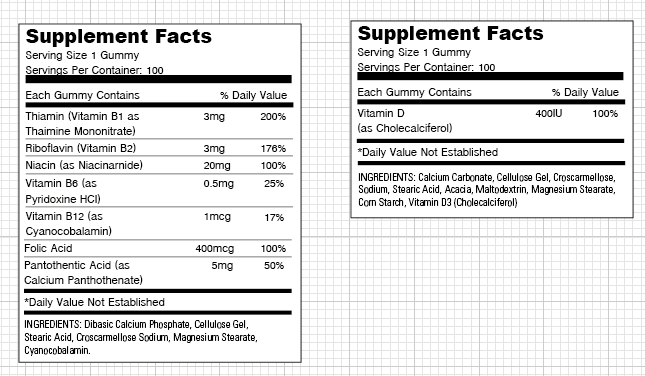The image is a large square with a grid-patterned background. It showcases two versions of a supplement facts label. The label on the left is a prominent rectangle occupying nearly the entire left side of the image. It features the bold text "Supplement Facts" at the top, with "Serving Size: 1 Gummy" written below in smaller black font. The label on the right is more compact, forming a square that only covers the top right quadrant of the image. This label also starts with "Serving Size: 1 Gummy," followed by the detailed supplement facts below.